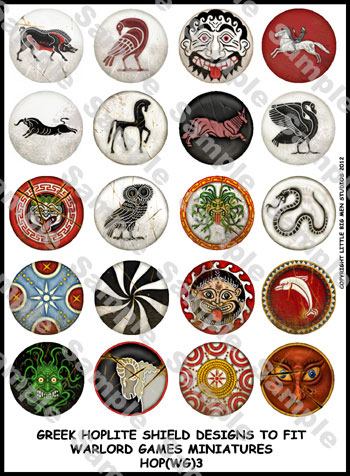The image is a photograph featuring a grid of circular shield designs intended for Warlord Games miniatures, specifically labeled at the bottom as "Greek hoplite shield designs to fit Warlord games miniatures, HOP(WG)3". The grid consists of four columns and five rows, making up a total of 20 distinct emblem designs. Each circle showcases varied imagery, primarily featuring animal motifs and mythological symbols. 

In detail, starting from the upper left:
1. A bull.
2. A red peacock.
3. A man with a clown-like face.
4. A white horse.
5. A white alligator.
6. A horse.
7. A black lion.
8. A goose with wings.
9. A red circle with a tiger-like face.
10. An owl.
11. A plant with a face.
12. A serpent.
13. A blue and red pattern.
14. A black and white peppermint swirl.
15. A cat face on a red and silver background.
16. A dolphin on a red background.
17. A green monster head.
18. A white unicorn.
19. A design with a yellow center and red semicircles.
20. Beady devil eyes in the bottom right-hand corner.

The image captures the intricate and diverse designs adorning these miniature shields, reflecting the rich variety of Greek hoplite insignia.